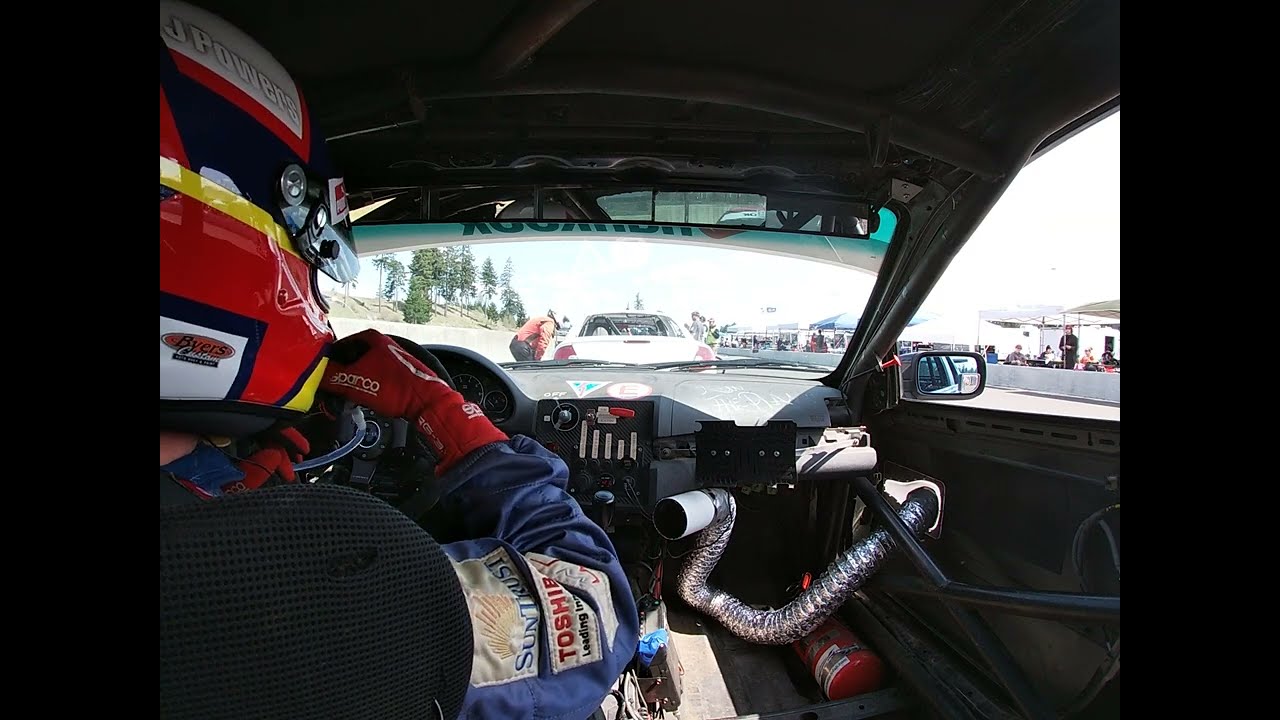The image captures the interior of a dilapidated race car from the perspective of someone sitting behind the driver's right shoulder. The driver, clad in a blue racing suit, red racing gloves, and a multicolored helmet featuring red, white, yellow, and black, grips the steering wheel with both hands. The car's interior is predominantly black, with its passenger side notably missing a seat. A silver, dryer vent-like hose snakes from the passenger door to the center console, ending at a spout. A red fire extinguisher is visible on the floor near where the passenger seat would be.

The dilapidation of the car is further emphasized by the rough and unfinished elements, including the makeshift hose setup. Out the front windshield, a white car is stopped in front, with what appears to be a police officer interrogating its driver. The background includes an overcast sky, trees on the left, and stands on the right with canopies sheltering onlookers, possibly race officials or the pit crew. A track banner is partially visible at the top of the windshield, and further beyond, the border of the racetrack and a hill with trees can be seen.

This detailed scene suggests a moment of preparation or a pause before a race, encapsulating the gritty, raw essence of racing.